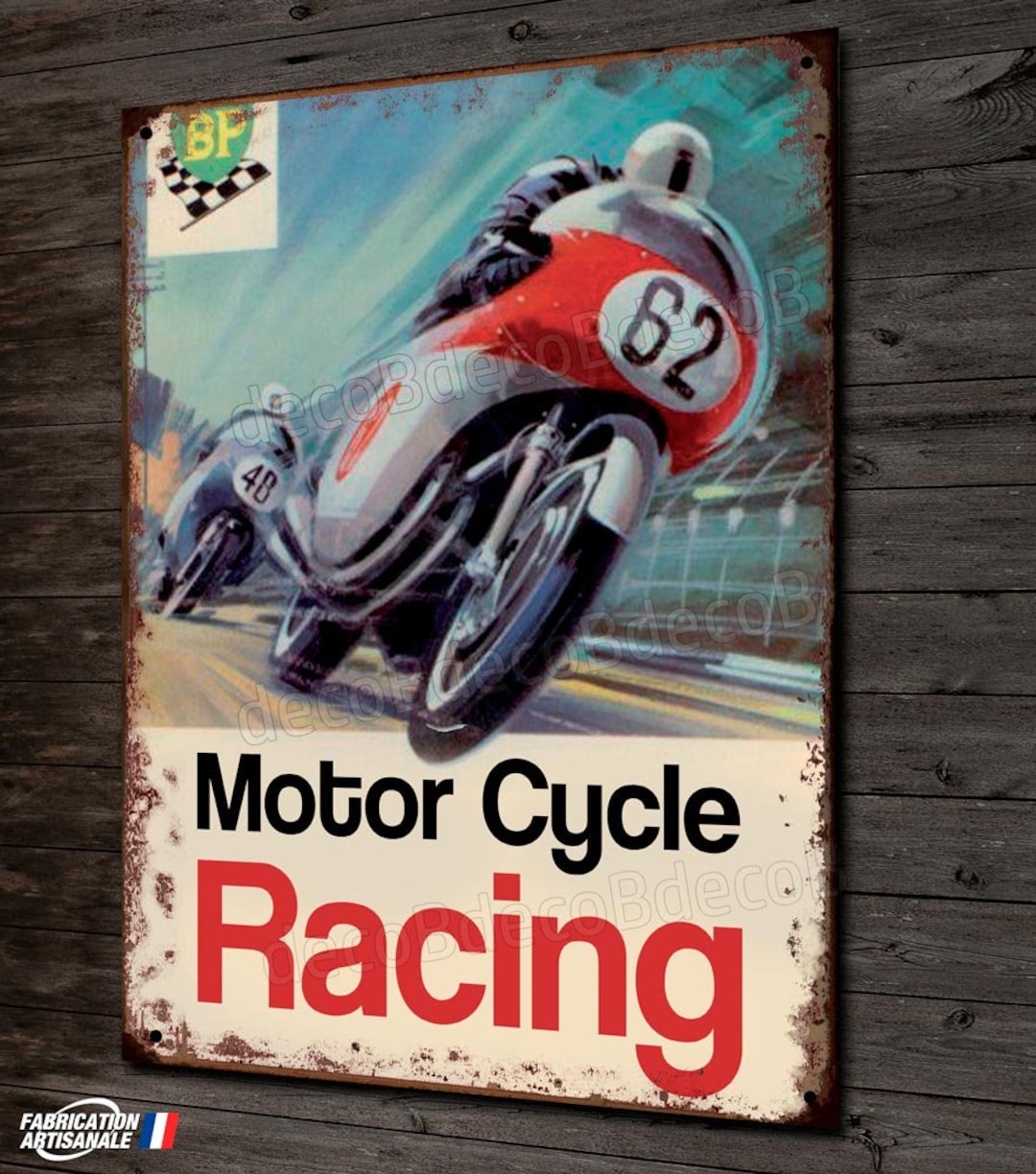The image features a vintage-style metal poster hanging on a dark gray wooden wall. The poster is weathered, with rusted edges and small holes at each corner, suggesting it was once used for public advertising. It prominently depicts an exhilarating motorcycle race with two futuristic, high-speed motorcycles. The leading motorcycle is red and white, bearing the number 62, while the second one is blue and numbered 48. Both riders are in full gear, complete with helmets and leather jackets, racing on what appears to be a professional track, indicated by the blurred speed lines and hints of a stadium on the right side of the image. At the bottom of the poster, "Motorcycle Racing" is boldly written, with "motorcycle" in black and "racing" in red against a tan background. In the upper left corner, there's a vintage British Petroleum (BP) logo featuring a green backdrop, yellow BP letters, and a black and white checkered flag. The bottom left corner highlights the name "Fabrication Artisanal San Ali" alongside a red, white, and blue striped flag.